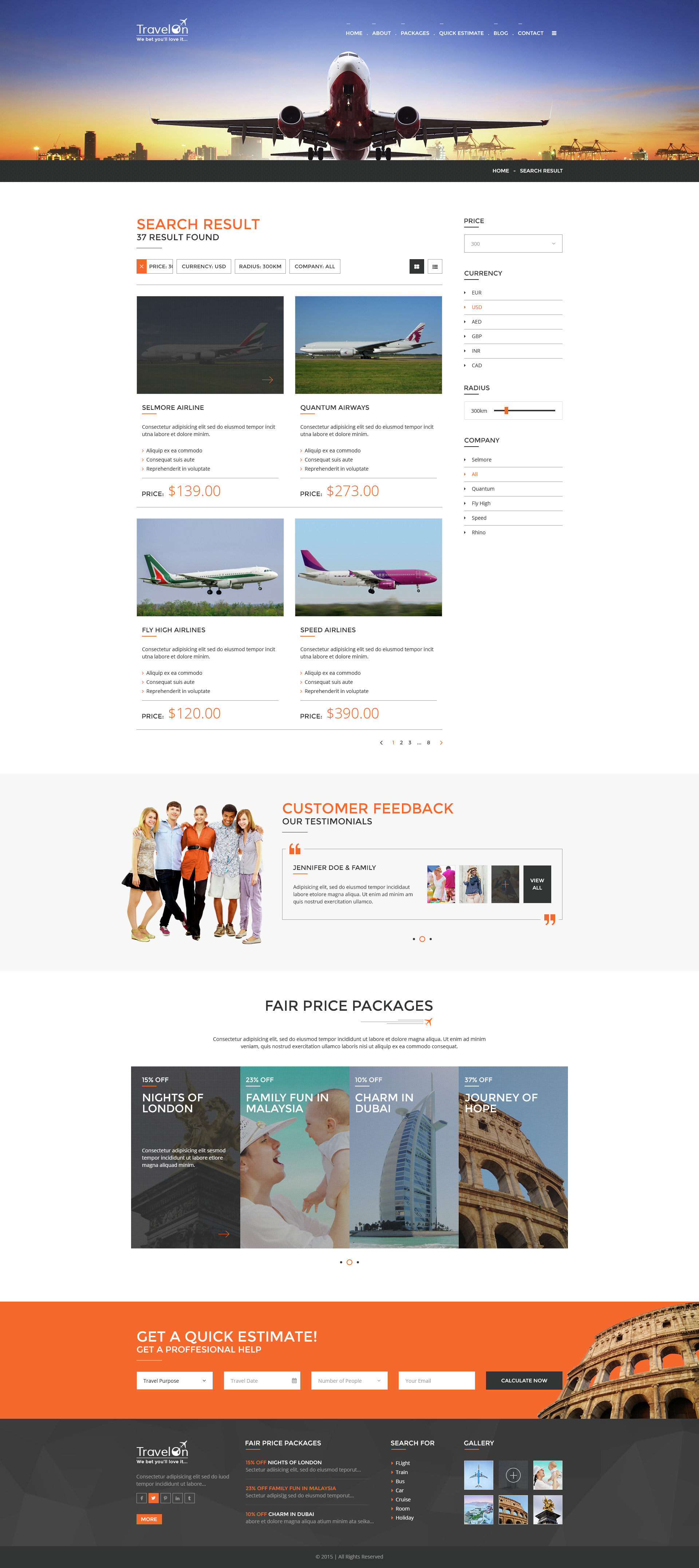The image appears to be a highly compressed, promotional graphic related to aviation, possibly for an airline or an airplane trading website. The overall theme combines elements of travel and commerce.

At the top of the image, there is a heading featuring a large airplane with either an airport or a cityscape in the backdrop. The scene is captured during twilight—either dawn or dusk—evident by the low light conditions and the positioning of the sun.

Below the heading, the phrase “Search Results” is prominently displayed in orange. Underneath this section, there are four thumbnails, each showcasing a different airplane with respective prices listed as $139, $273, $120, and $390. This suggests that the site may be involved in buying or selling planes.

Further down, there is a light blue box intended for customer feedback. Within this box, five individuals stand side by side with their arms around one another, accompanied by a customer testimonial to their right, though the text is unreadable.

The section titled "Fair Price Packages" follows, featuring four additional thumbnails. The images include a person holding a baby, a peculiar building, and the iconic Colosseum. However, the text associated with these images is not legible.

At the bottom of the image, there is a two-tone section: the top part is orange and the bottom part is black. This area includes a call to action titled “Get a Quick Estimate.” It features four text input boxes, though their labels are not readable. To the right of these boxes, there’s another image of the Colosseum, with a series of clickable elements and six small thumbnails at the very bottom.

Overall, the design aims to attract users interested in aviation, offering information about airplane transactions and travel packages, although the legibility of specific details is impaired by compression.